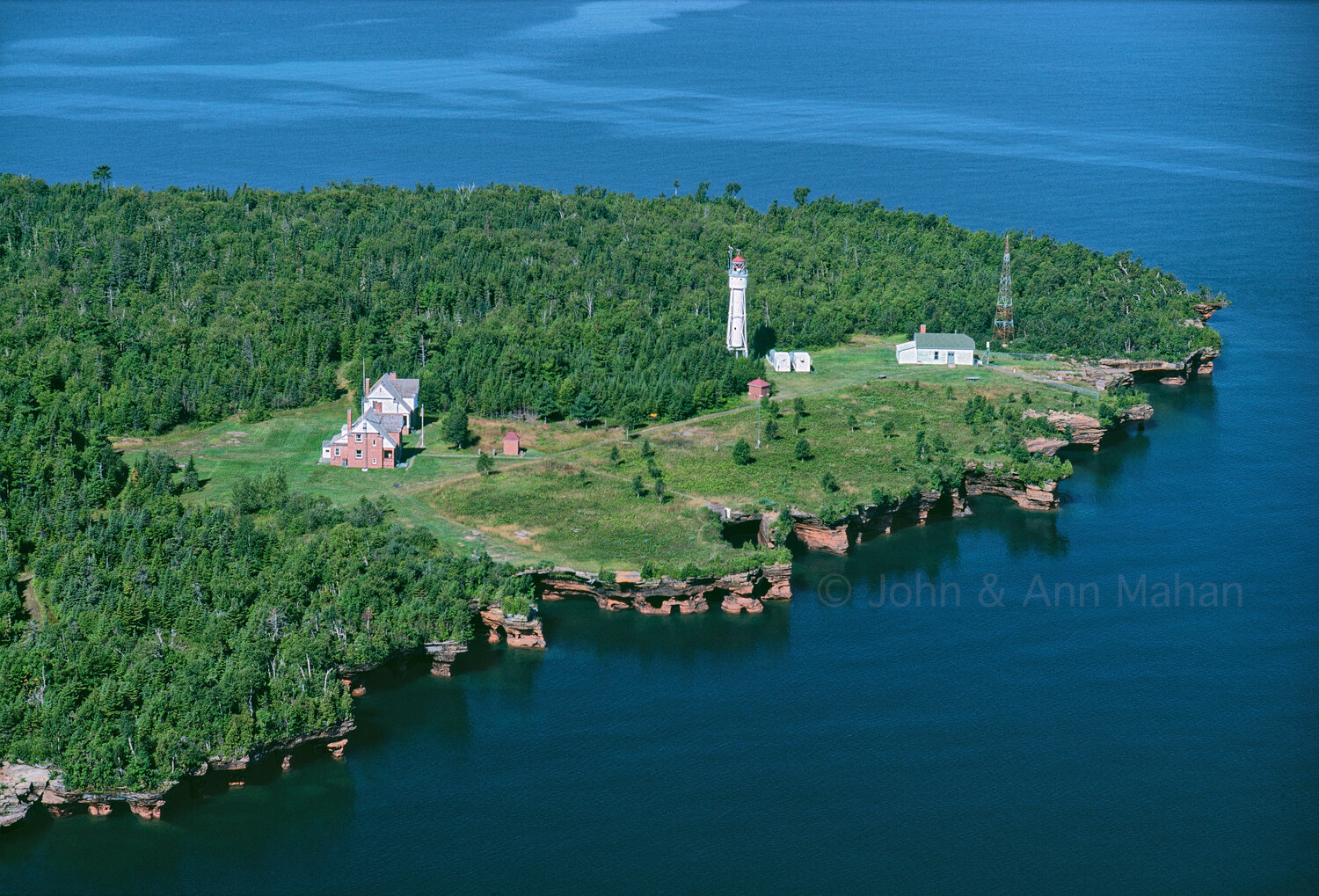The image presents an aerial view of a pointed landform, either an island or a peninsula, extending from the middle left to the middle right of the frame, and narrowing to a point. The foreground reveals the rugged shoreline composed of layers of red rock crowned with lush green grass and forests. To the left, two houses can be seen: one is red-brick with a white roof, and next to it, another house with similar architecture but featuring white walls. Further towards the water on the right side lies a shed with a green roof adjacent to a solitary lighthouse. A tall radio tower is positioned to the right of the shed, indicating some form of signal transmission. The background is dominated by endless green trees, with the calm blue ocean surrounding the land. The text "copyright Jonan" is prominently displayed, with a mention of "Mahan." The diverse color palette includes ocean blue, various shades of green, red brick, grayish beige, and white.